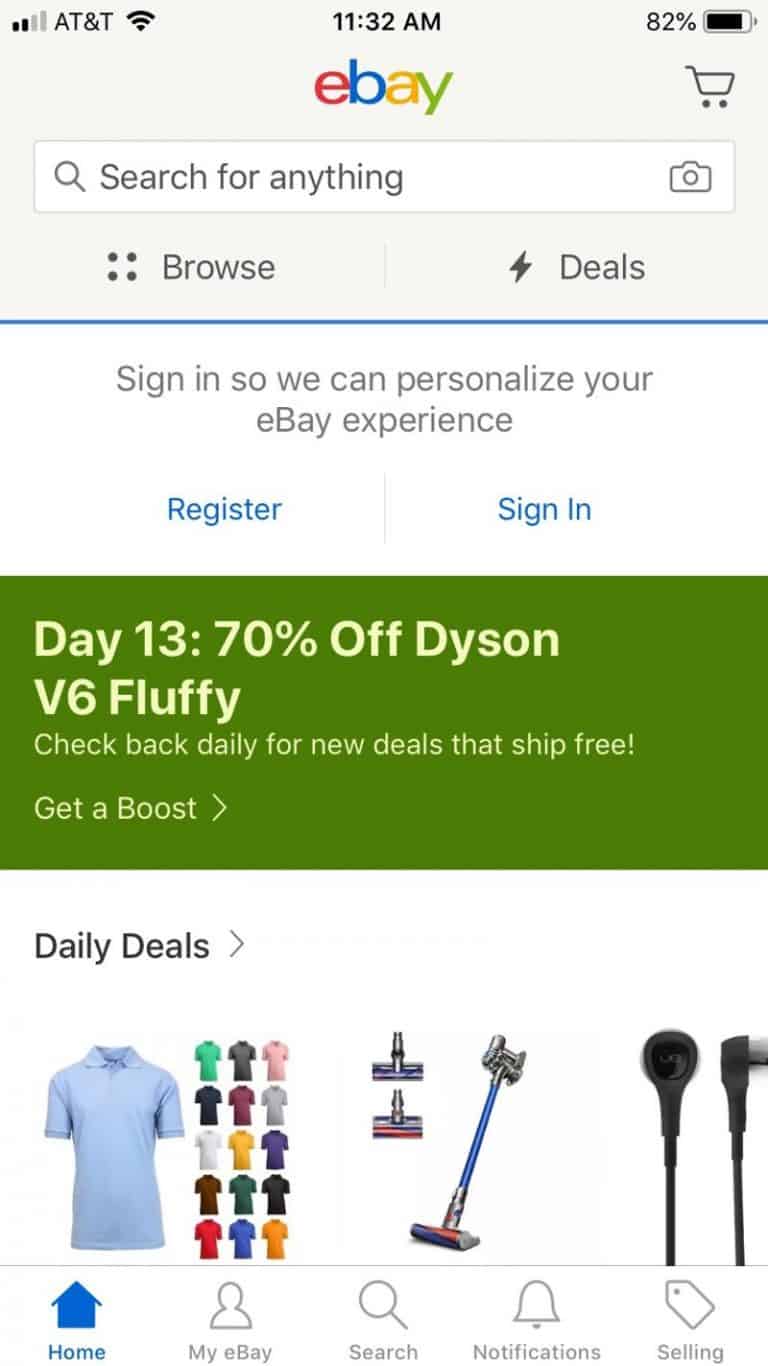In the image, a smartphone screen displays the eBay app interface. At the top left, the screen shows the AT&T network connection and a Wi-Fi icon, indicating the device is connected to the internet. The middle of this section shows the current time, 11:32 AM, while the battery percentage is displayed at 82% on the right.

Just below, the eBay app UI starts with the eBay brand name and a shopping cart icon to its right. Beneath these is a white search bar labeled "Search for anything." Next, a row includes the "Browse" and "Deals" tabs, followed by a prompt to sign in for a personalized experience. Below that are two buttons: "Register" on the left and "Sign in" on the right.

Further down, there's a promotional banner in a green rectangle reading "Day 13: 70% off Dyson V6 Fluffy. Check back daily for new deals that ship free. Get a boost." Underneath this banner, "Daily Deals" is written in black. The main content includes images of various products: starting from the left, a large blue shirt, followed by five rows of three smaller shirts in different colors. To the right is an image of vacuums or mops, and next to that, a pair of headphones.

At the bottom, the navigation bar consists of five icons from left to right: "Home" (highlighted in blue), "My eBay," "Search," "Notifications," and "Selling" (all gray). This completes the layout of the displayed eBay app screen.